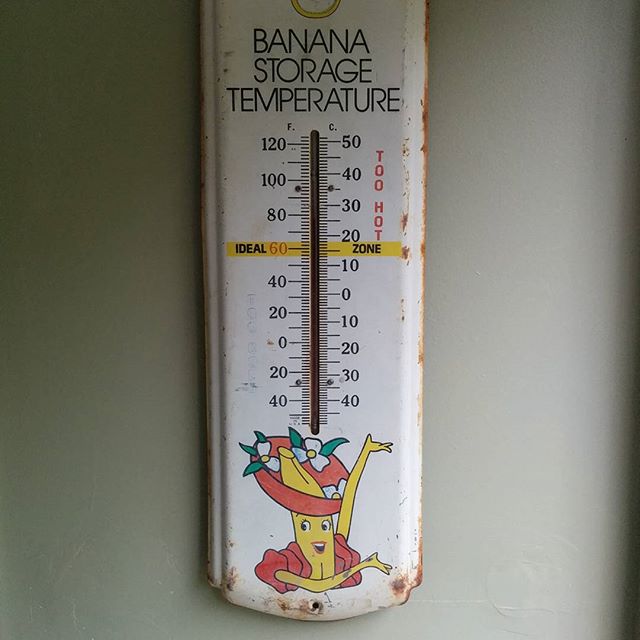A square image showcases an outdoor wall with an attached, heavily weathered thermometer. The wall has an olive-green hue, which appears more pronounced on the left side and lightens to a grayish tone on the right. The thermometer, positioned almost centrally from top to bottom, is painted white and made of heavy aluminum. Its age is evident from the significant rust, particularly on the right side, likely caused by prolonged exposure to rain.

At the top center of the thermometer is a small yellow half-circle with the inscription "Banana Storage Temperature" below it, suggesting it is designed to help store bananas at an optimal temperature. 

The thermometer features two temperature scales. On the left, the Fahrenheit scale ranges from 120°F to -40°F, with an "Ideal" indicator marked in yellow at 60°F. The right column shows the Celsius scale, marked from 50°C to -40°C, with "Too Hot" and "Ideal Zone" indicators in red and yellow respectively. The ideal temperature for banana storage on the Celsius scale is around 15°C, correlating with 60°F on the Fahrenheit side.

At the bottom, there is a graphic resembling the Chiquita bananas logo: a large yellow banana with a red hat adorned with white petals and big fluffy red sleeves, giving the thermometer a touch of whimsy and branding.